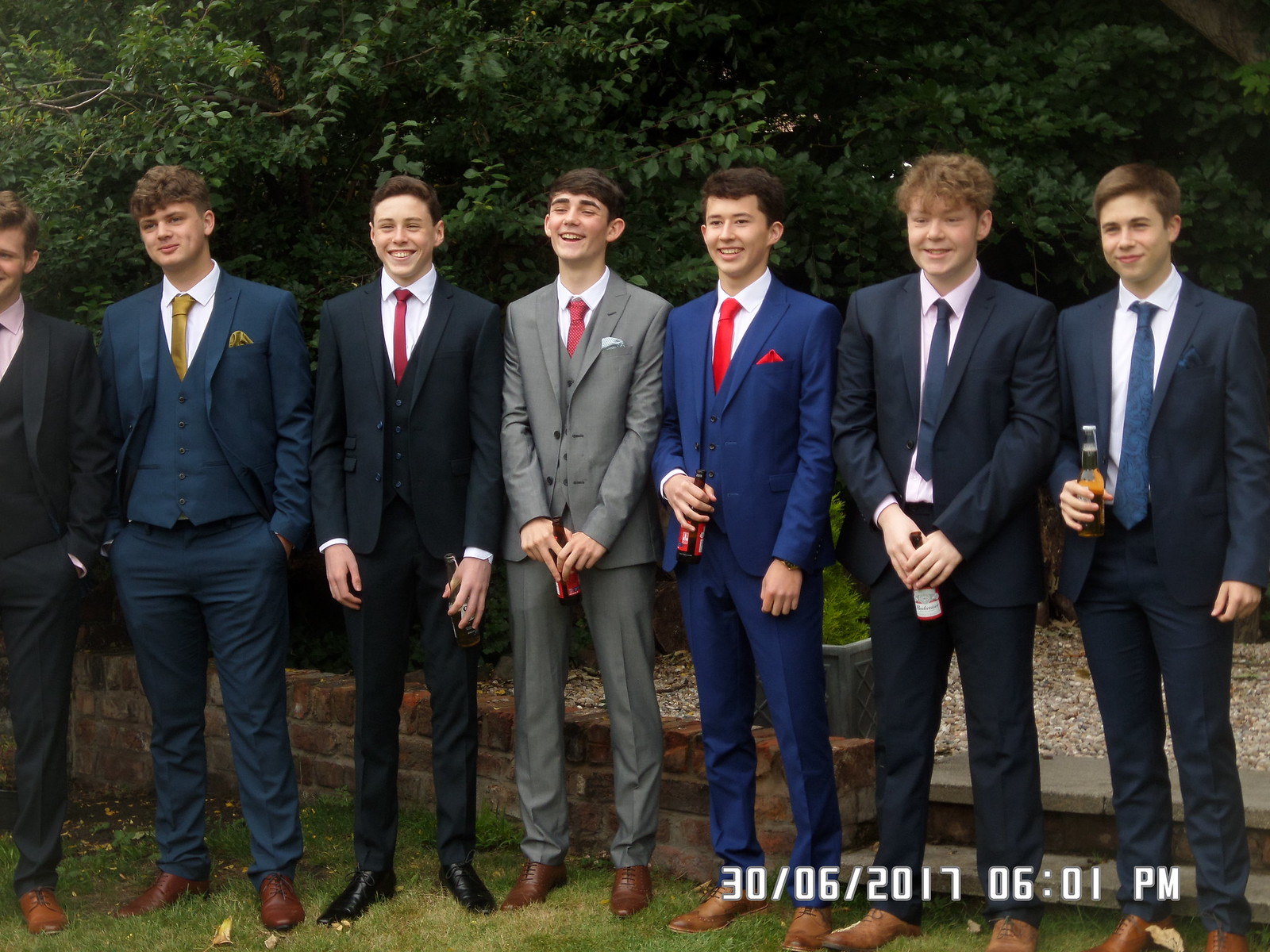The image depicts seven young men standing in a line, all dressed in suits with a variety of colored ties and shoes. The young men, all smiling with short brown hair, are wearing either blue, black, or gray suits, and they stand against a backdrop of deciduous foliage. Four hold beer bottles, with one identifiable as Budweiser; detailed labels on the other bottles are not clear. Specifically, the boys on the far left and right are wearing blue suits, while the central figure in a gray suit is flanked by one person in a black suit on his left and another in a light blue suit on his right. The text at the bottom right corner of the photograph reads "30-06-2017 06:01 p.m."